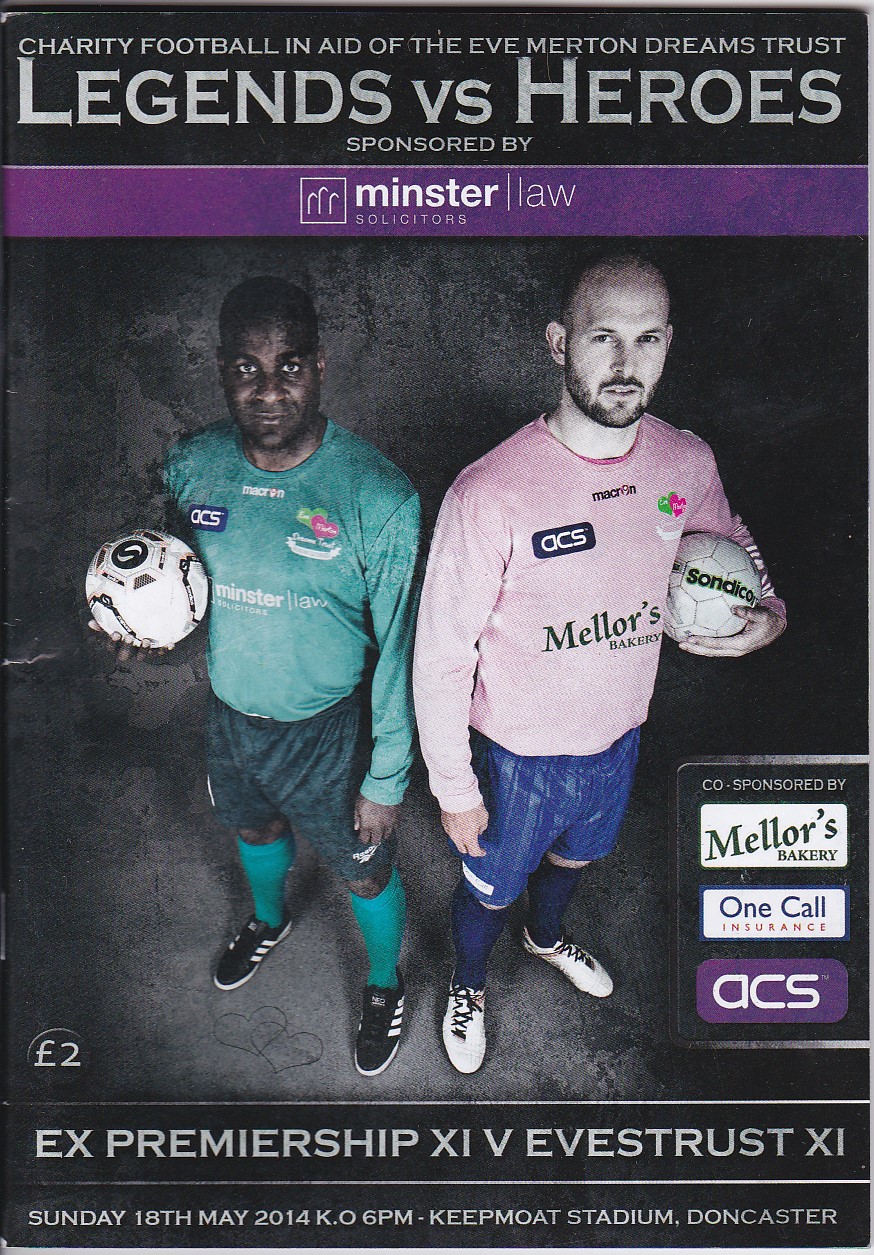The magazine cover is dedicated to an advertising event poster for a charity football match in aid of the Eve Merton Dreams Trust. At the top, in silver font, it reads "Charity Football in Aid of the Eve Merton Dreams Trust." Below this, a purple banner with white font displays the text "Minster Law Solicitors."

The focal point of the cover features two men holding soccer balls. On the left is an African American man wearing a complete green football kit from Minster Law Solicitors, including a long sleeve green jersey, dark green shorts, and tall green socks, paired with black shoes that have white bottoms and stripes. He is holding a white soccer ball in his right hand.

To his right stands a Caucasian man wearing a long sleeve pink soccer jersey emblazoned with "Mellor's Bakery." He has blue shorts, blue socks, and white shoes. He is holding a soccer ball marked with "Saunders" in his left hand. This man has both a mustache and the beginnings of a beard.

Additional information at the bottom of the poster includes the match details: "Ex Premiership 6 vs. Evastrust 11, Sunday the 18th of May 2014, K-O 6 p.m., Keep Moat Stadium, Doncaster." Sponsorship mentions from Mellor's Bakery, One Call Insurance, and ACS appear on the side.